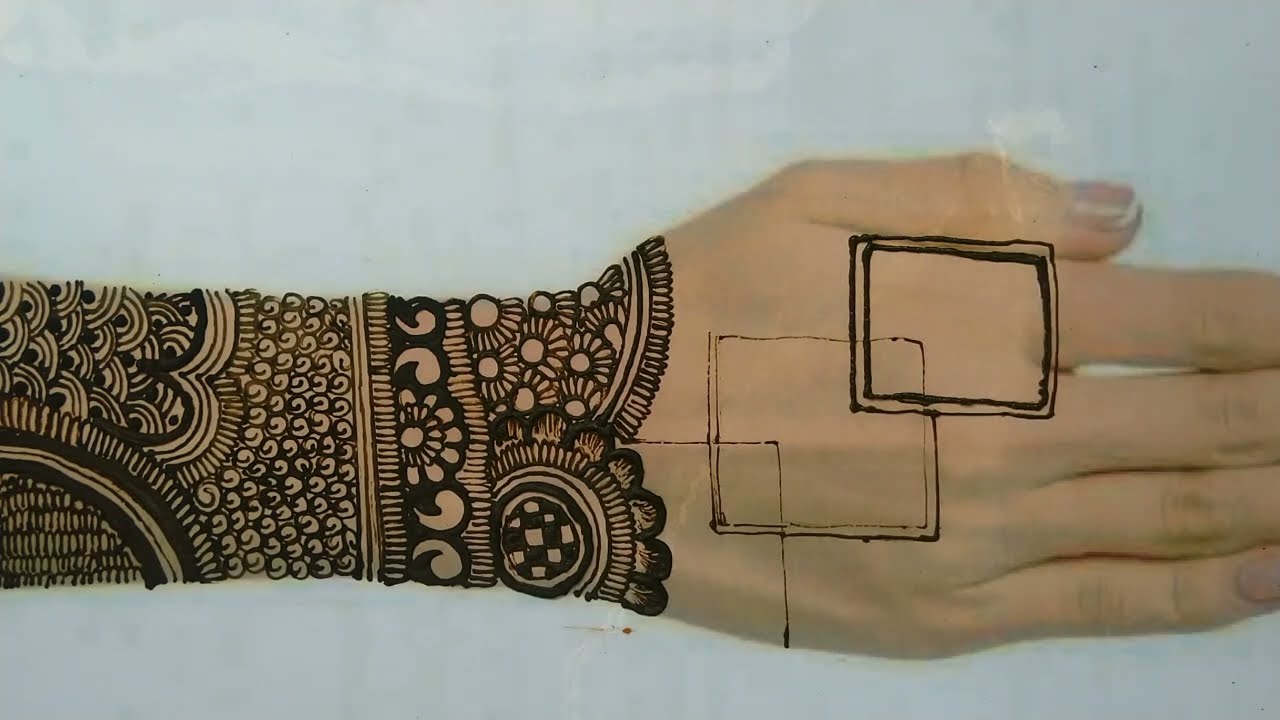In this rectangular image, approximately six inches wide and three inches tall, we see a close-up, detailed photograph of a Caucasian person's right forearm and hand placed against a light blue background, which could be a bedsheet. The forearm extends from the center left to the center right, with the tips of the index, middle, and ring fingers partially cut off at the edge of the image. The pinky fingernail and thumbnail are both visible. The skin tones in the image range from tan to light brown.

The forearm is adorned with an intricate henna tattoo featuring geometric designs. These details start with small, round shapes and extend towards the hand, where the design transitions into various square patterns. On the hand itself, the topmost square on the wrist shows a double square (a square within a square), the middle square is partially outlined with a similar double-layering effect, and at the bottom left of the hand, there is a partial square due to space constraints. The overall detailed decoration showcases the complexity and beauty of henna art, adding a cultural and artistic depth to the image.